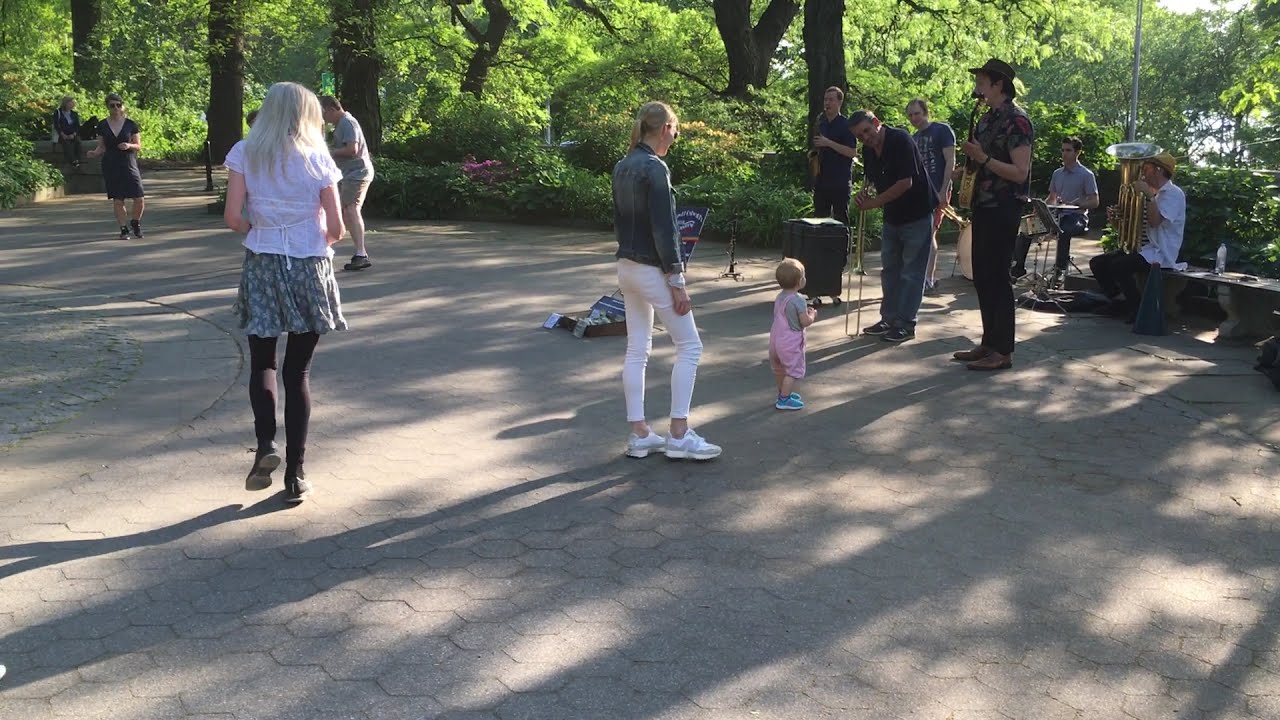In a sun-dappled, shaded stone plaza within a verdant park, a lively scene unfolds featuring a six-piece street performing band. Positioned towards the upper right corner of the horizontal image, the musicians include a saxophonist, a trombonist, a tuba player, a guitarist, and a drummer, accompanied by another member whose instrument is indiscernible. The band is busily entertaining a small crowd.

Central to the scene is a woman dressed in a denim shirt or jacket, white pants, and white shoes, standing protectively behind a toddler in pink overalls and blue shoes. The child gazes up in awe at the musicians, tentatively moving closer to the tempting melodies. The mother observes with a relaxed posture, ensuring the safety of her curious child.

To the left, various park goers stroll casually, adding to the atmosphere of leisurely enjoyment. The broad concrete pavement spans much of the lower portion of the image, forming the stage where life's everyday moments play out. The background is lush with greenery, punctuated by the dark trunks of mature trees, and possibly a serene lake, all under a bright daytime sky. An ambient speckling of sunlight penetrates through the foliage, casting playful shadows and highlighting the conviviality of the setting.